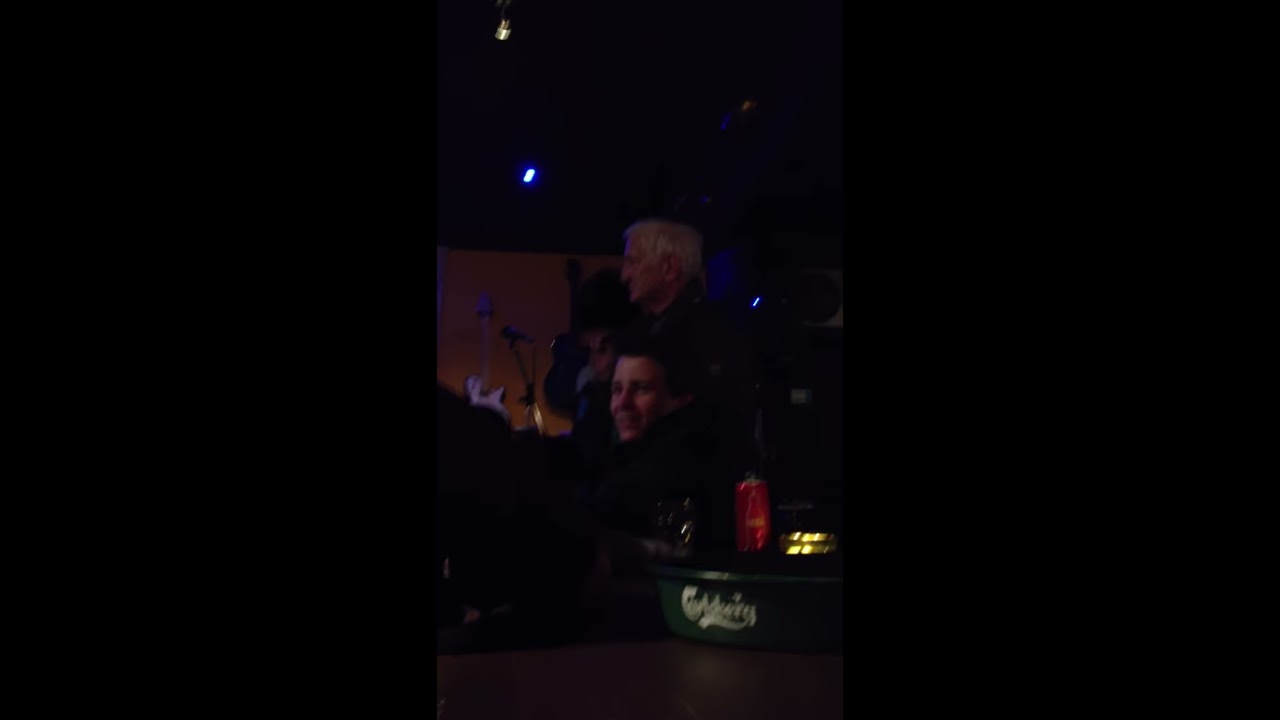In this indoor scene, possibly at a nightclub or concert venue, the image captures two individuals' left side profiles prominently in the center. An elderly man with white hair, potentially in his 70s, is positioned above a younger, androgynous individual with short, dark hair. The dimly lit setting is characterized by contrasting light sources: a blue and a yellowish light from above. 

Behind the younger figure's back and shoulder, a red Coca-Cola can is noticeable, next to a container or ashtray bearing illegible white text. The environment suggests a musical ambiance, with an electric guitar propped against a brown panel and a microphone visible in the background. The vertical cell phone photograph is extremely dark and blurry, highlighting a black background on either side, an unfinished ceiling, and isolated lit areas that heighten the room's overall dimness.